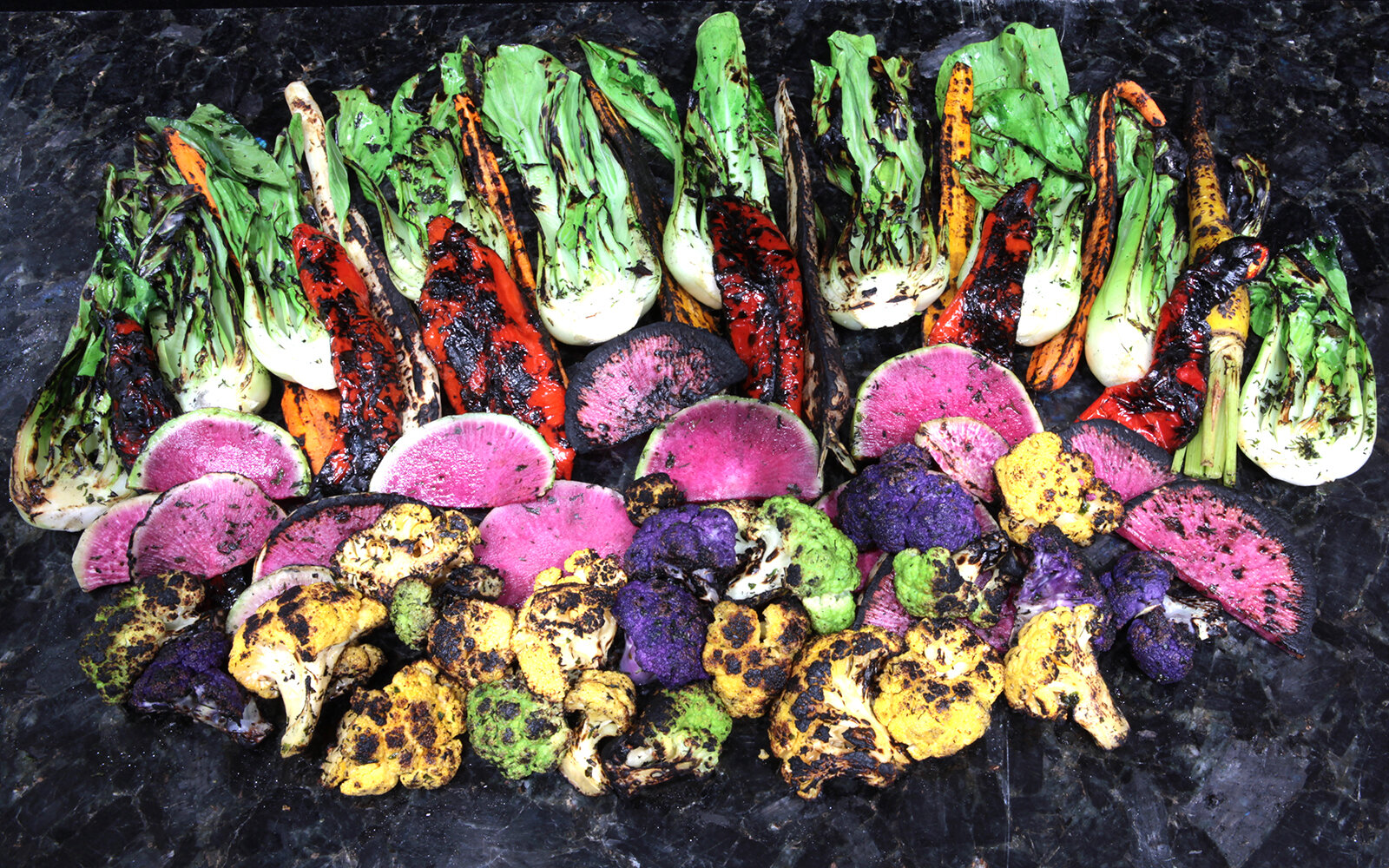This photograph showcases a vibrant and somewhat surreal arrangement of various charred vegetables, set against an almost black, charred background that resembles charcoal. The photo composition places an emphasis on the vivid hues of the vegetables, which appear partially grilled, imparting a blackened, smoky texture. At the top, there are several light and dark green leafy vegetables, possibly bok choy or a form of grilled cabbage. Among these are large charred red and orange peppers, interspersed with lighter yellow and orange carrots.

As the eye moves downward, you encounter an assortment of cruciferous vegetables—broccoli, cauliflower, and unique purple broccoli. These too bear the distinct marks of grilling, their colors ranging from typical green and white to more unusual yellow and purple shades. There's also mention of fruits with a striking appearance, such as half-circle slices that are pink-red with white edges, possibly hinting at something akin to watermelon, though they also show signs of charring.

The whole arrangement is laid out in an almost random, yet visually striking order, making the photograph both a feast for the eyes and a curious composition of grilled produce. The overall effect is emphasized by the stark contrast between the vegetables' bright colors and the dark, ash-like background, creating a dynamic and captivating piece.